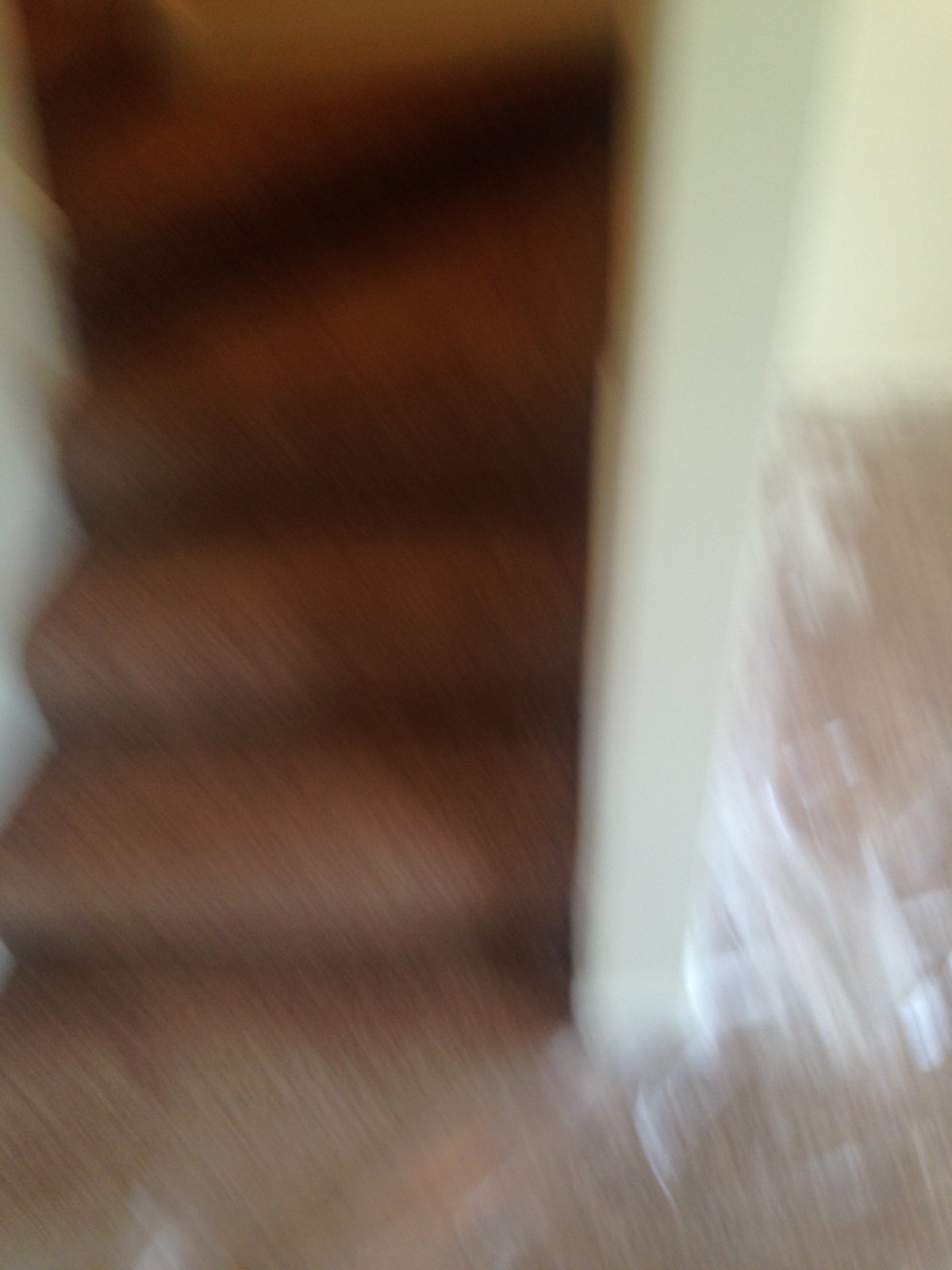The photograph depicts a blurry interior shot of a home, characterized by a somewhat indistinct, yet intriguing atmosphere. In the lower right corner, there's an object that appears to be wrapped in shiny plastic, possibly a box or a package that has yet to be opened. The floor is carpeted in a light grayish hue, which extends to a visible stairwell comprising at least four carpeted steps. Despite the blur, the lighting within the room is decent, offering a warm and inviting glimpse into this somewhat mysterious domestic scene.